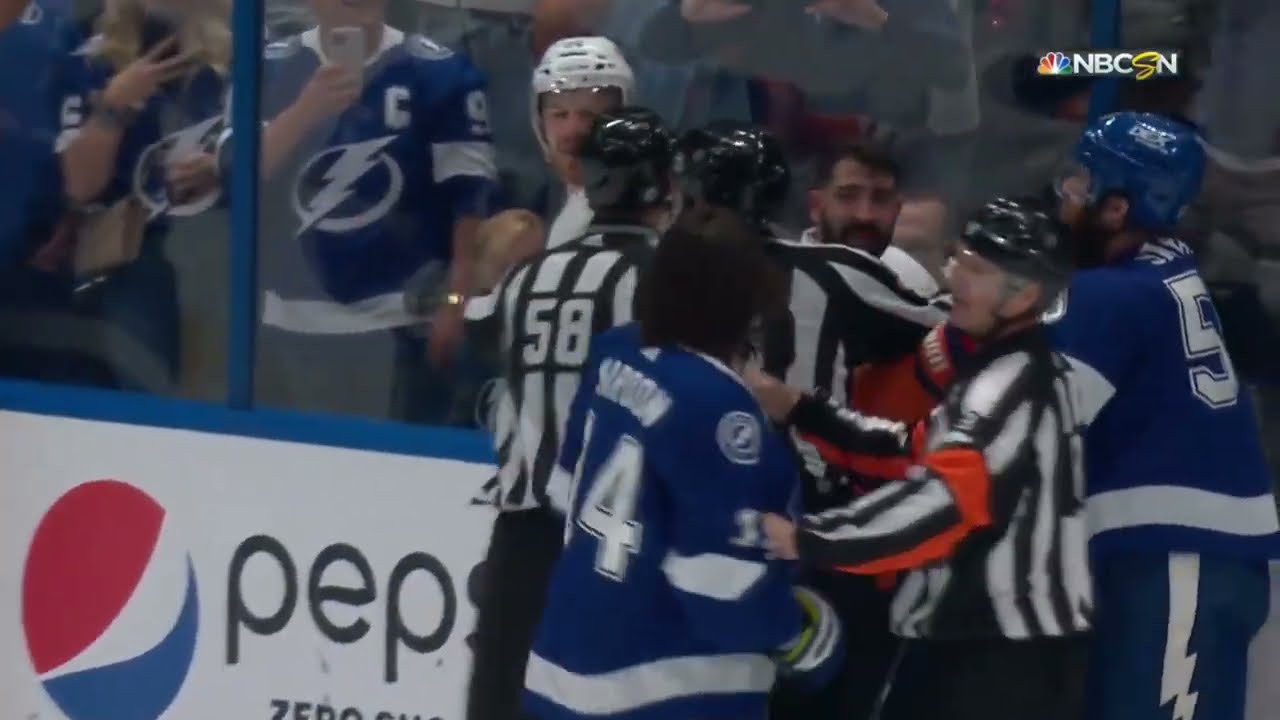The image captures an intense moment in a hockey game, prominently displaying several players in blue jerseys with white lettering and a distinct white band around the waist, and blue pants with a white stripe down the side. The scene is centered on a heated skirmish being broken up by three referees dressed in black-and-white striped shirts, black pants, and helmets. Referee number 58 is discernible, along with another referee who has a red band tied around his arm. Among the players, two wearing blue-and-white jerseys appear to be the main combatants, with another player in a white helmet nearby. Behind them, a white barricade featuring a prominent Pepsi Zero Calorie advertisement separates the action from the glass partition. Beyond the glass, a captivated crowd of fans, some donning jerseys emblazoned with a lightning bolt logo, can be seen, and one person is notably capturing the event on video. The upper right-hand corner of the image bears the NBC logo, indicating this is likely a high-definition screenshot from a televised broadcast.